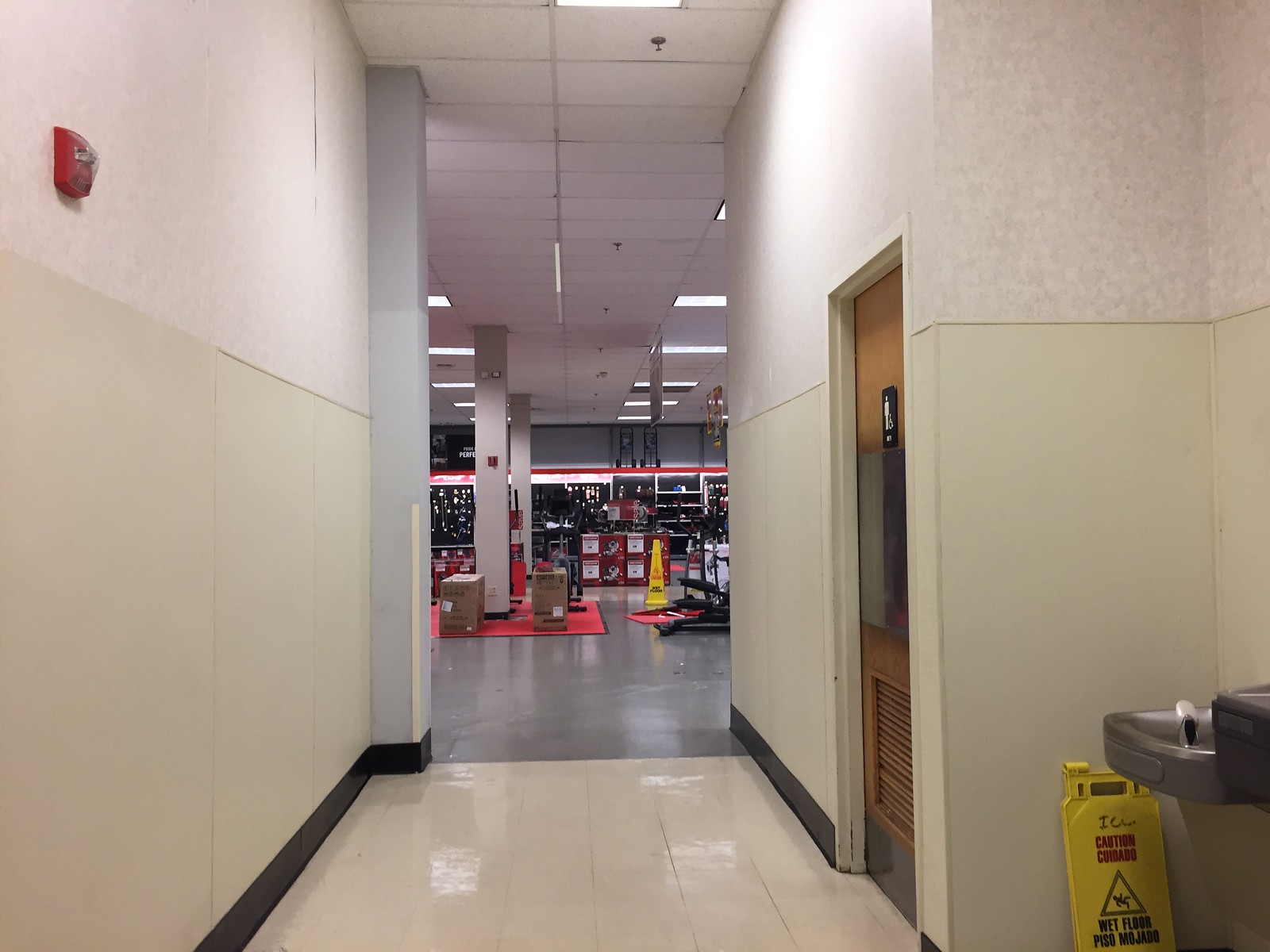This photograph depicts a well-lit hallway in a department store, extending into the main shopping area. The hallway features a cream-to-white gradient wall with a red, square-shaped fire alarm on the left side. The fire alarm has a curved, clear top section with a small metal piece inside for activation. The floor is white tile, separated into small squares without visible grout, and the baseboard at floor level is painted black. A dark gray pillar stands on the left side, while the ceiling consists of white rectilinear drop ceiling tiles interspersed with gray sprinkler heads and numerous fluorescent lights.

On the right side of the hallway, there is a brown door marked with a handicap accessible symbol, a silhouette of a person, and a wheelchair silhouette, accompanied by a slightly blurred gray box above the signage. The door has a dark gray metal sheet with ventilation at the bottom. A silver and dark gray water fountain stands in the right-hand corner, next to a folded caution sign in yellow warning of a wet floor in both English and Spanish, with an image of a falling person in a triangle.

Looking into the store from the hallway, the shop space transitions from the white tile to a dark gray, possibly concrete, floor. Visible within the store area are white and dark gray pillars, black wall-mounted tools, red cardboard boxes, and shelves. Banners, likely indicating sales or clearance, hang from the ceiling. An additional red rug is visible with various items on it, and there is another yellow caution sign indicating a wet floor. The overall color palette in the image includes red, white, gray, black, and yellow.